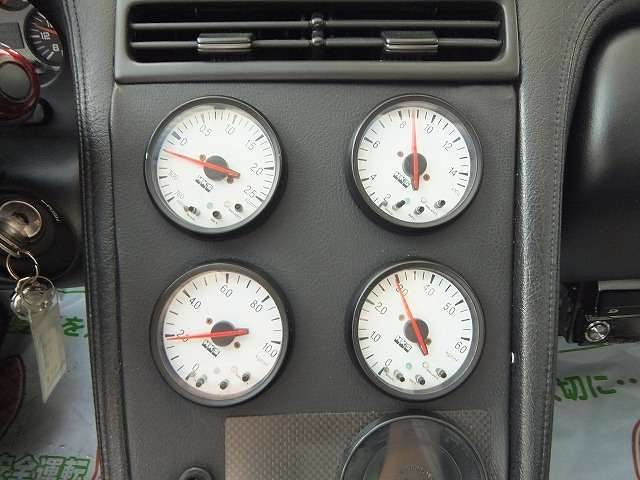This photograph captures the console area of the dashboard of a seemingly sporty vehicle, characterized by its array of analog dials dedicated to various engine functions. Notably, the specific functions of these dials—potentially including vacuum pressure, oil pressure, and temperature—are not explicitly labeled. Instead, the driver must be familiar with each gauge and its corresponding function.

The dials are uniquely mounted at an angle, ensuring that the zero position points directly towards the driver, while the 12 o'clock position points away. This innovative orientation allows the driver to quickly glance down and confirm that all indicators are pointing upward, akin to the setup in professional race cars, signifying optimal engine performance.

Adding to the vehicle's vintage and sporty charm, the keys are inserted into an old-fashioned ignition. On the floor mats, there are what appears to be Japanese characters, suggesting that the vehicle is of Japanese origin, though the symbols could also be Korean.

Additionally, in the upper left corner of the dashboard, more analog dials are visible. The photograph also captures the top of an air conditioning and heating vent, completing the detailed view of this sporty, possibly Japanese-made vehicle's dashboard.